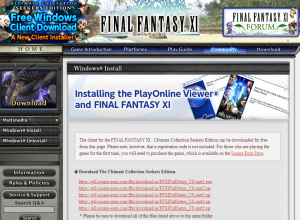The image showcases a comprehensive website interface dedicated to Final Fantasy XI. Prominently displayed at the top is the title "Final Fantasy XI". To the left of this title, there is a key feature: a "Free Windows Client Download" section, which offers a new client installer for the game. Additionally, the interface includes several navigational links such as "Installing the PlayOnline Viewer", "Final Fantasy XI", "Final Fantasy XI Forum", "Play Guide", "Download", and "Game Installation". The overall design of the website features a vibrant and striking color palette that includes black, red, brown, blue, yellow, orange, and green, contributing to an engaging visual experience.